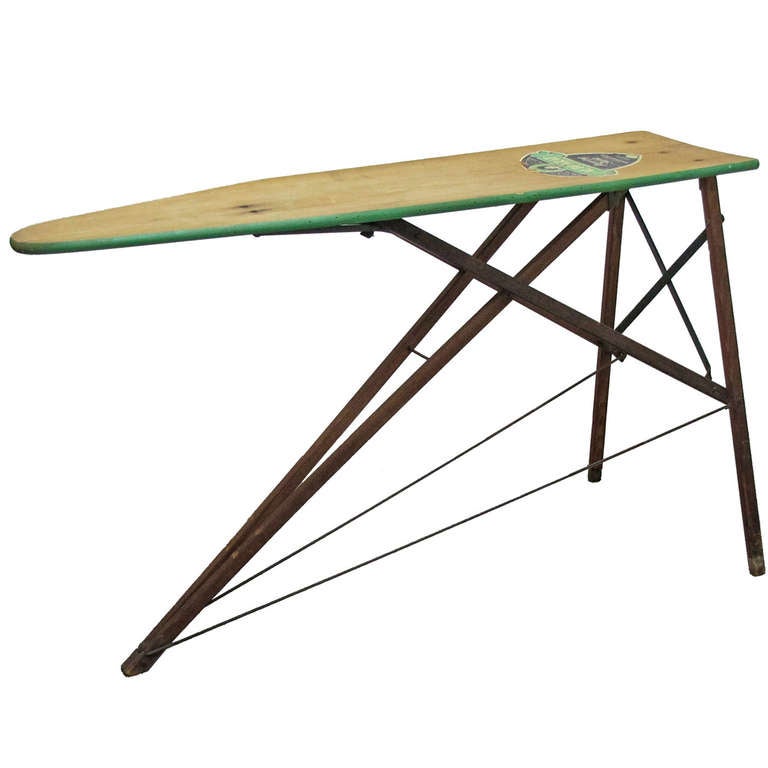This detailed color photograph showcases a vintage wooden ironing board with exposed steel folding legs. The ironing board top is constructed from wood and features three visible nail holes toward the front and additional nail holes at the rounded back end. Encircling the board is a green, felt-like border, adding a touch of texture. Near the back, a green and purple logo is visible, though its precise details are unclear. The board is supported by a set of steel legs, prominently showing some signs of rust. The rear legs have a supporting beam extending towards the front of the board, ensuring stability. The overall structure is designed with one pair of legs descending directly to the floor, while the other set extends forward, allowing for easy folding and setup.